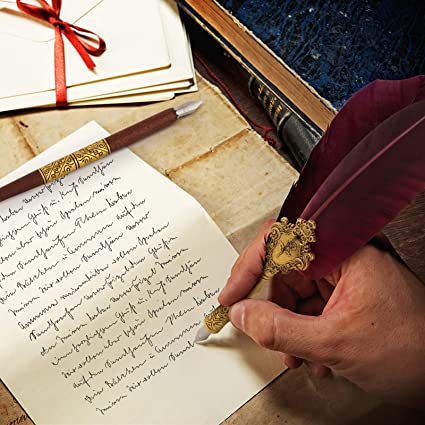The image depicts a close-up of a person's right hand, likely a man's, writing a letter with a luxurious quill pen. The pen features a smooth, maroon feather meticulously trimmed and shaped, attached to a gold embellished body with a silver tip, resembling a traditional dip pen. The individual is writing in an elegant cursive script on a cream-colored piece of paper, nearly filling the page with flowing black ink. Alongside the writing hand, situated towards the top of the paper, lies another unused quill pen, which is wooden with gold inlay.

In the background, neatly tied with a red ribbon, is a stack of beige envelopes. To the right of the writing hand, there are several old books, with one distinctly having a black cover and spine. The setting is a light brown wooden desk, creating a vintage atmosphere suited for an advertisement of calligraphy pens or stationary.